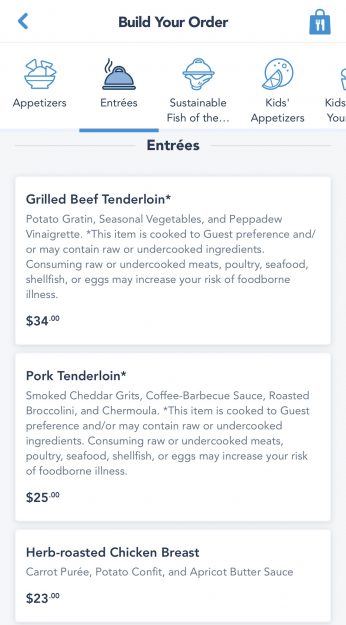This image is a mobile screenshot in portrait mode, featuring a menu interface. The layout is in a single column format, starting with a navigation row at the top. 

In the upper left corner, there's a blue back arrow, while the upper center displays "Build Your Order" in bold lettering. The upper right corner features a shopping bag icon containing utensils. 

The second row shows a series of category icons: Appetizers, Entrees, Sustainable Fish of the, Kids Appetizers, and Kids Cutoff. The "Entrees" category is highlighted in blue and underlined, indicating it’s the currently selected section.

Below this, a gray background row prominently displays "ENTREES" in bold, capital letters. 

The menu lists three entrée options with detailed descriptions:
1. **Grilled Beef Tenderloin** - Priced at $34, this dish includes potato gratin, seasonal vegetables, and peppadew vinaigrette. A note warns that the item is cooked to guest preference and may include raw or undercooked ingredients, which could increase the risk of foodborne illnesses.
2. **Pork Tenderloin** - Priced at $25, the pork is served with smoked cheddar grits, coffee barbecue sauce, roasted broccolini, and chermoula. It also carries the raw/undercooked ingredients warning.
3. **Herb Roasted Chicken Breast** - Priced at $23, this dish features carrot puree, potato confit, and apricot butter sauce.

Each entrée comes with its own set of accompaniments, enhancing the dining experience with unique flavor profiles and presentations.